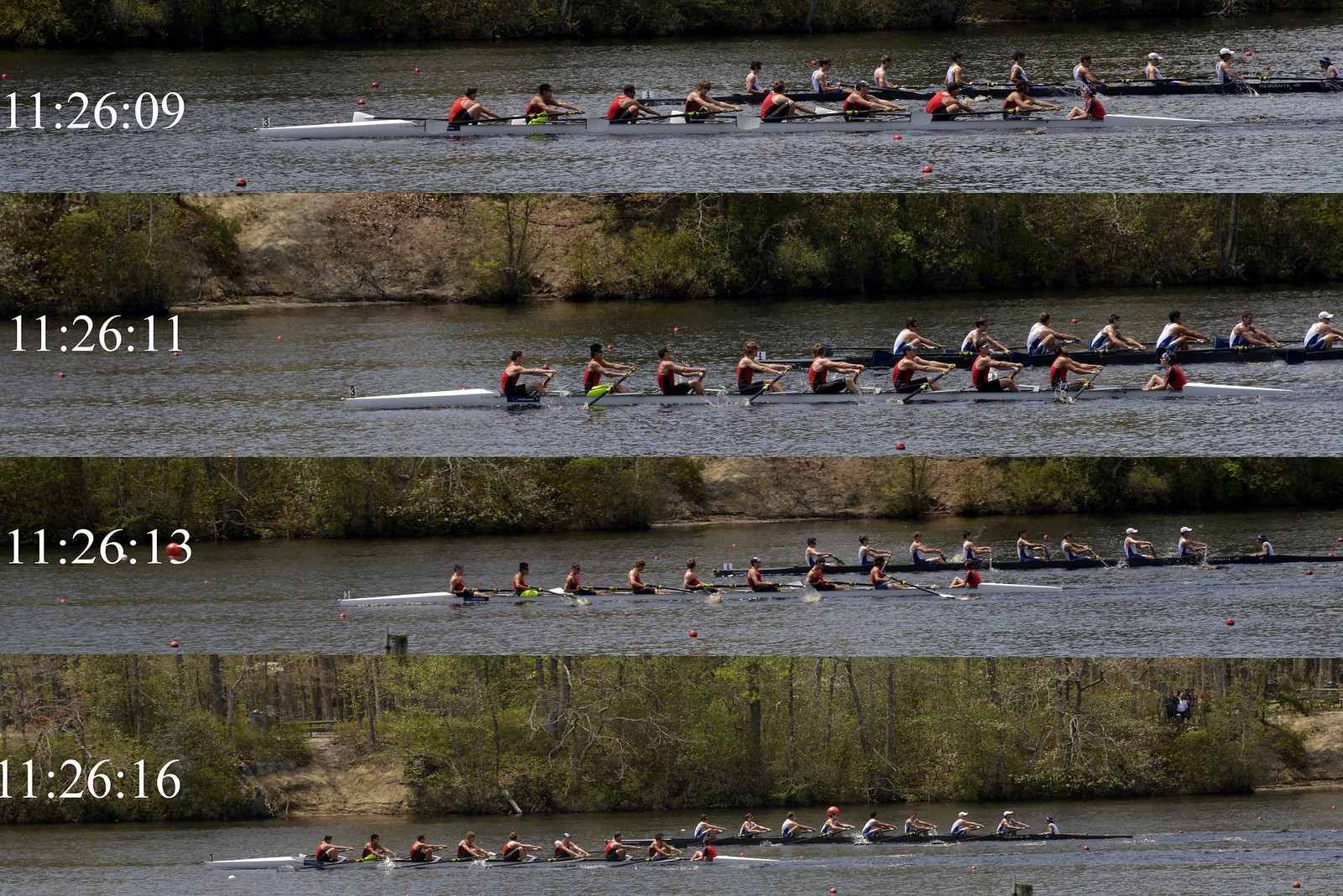The image consists of four vertically stacked photographs, each displaying a different time frame of a rowing race, emphasizing the progression of the event. To the left of each photograph is a timestamp: 11:26:09, 11:26:11, 11:26:13, and 11:26:16, indicating the moments captured. In each frame, two long, sleek racing boats, crewed by nine rowers each, can be seen racing on a dark-colored river. The crews are distinguishable by their uniforms; one team is dressed in red tops while the other wears white tops. The background of the images includes a dense forest with a variety of khaki and dark green shrubs and leaves visible along the riverbank. The sequence of photographs captures the continuous movement and changing positions of both boats as they navigate the water, providing a dynamic view of the rowing competition.